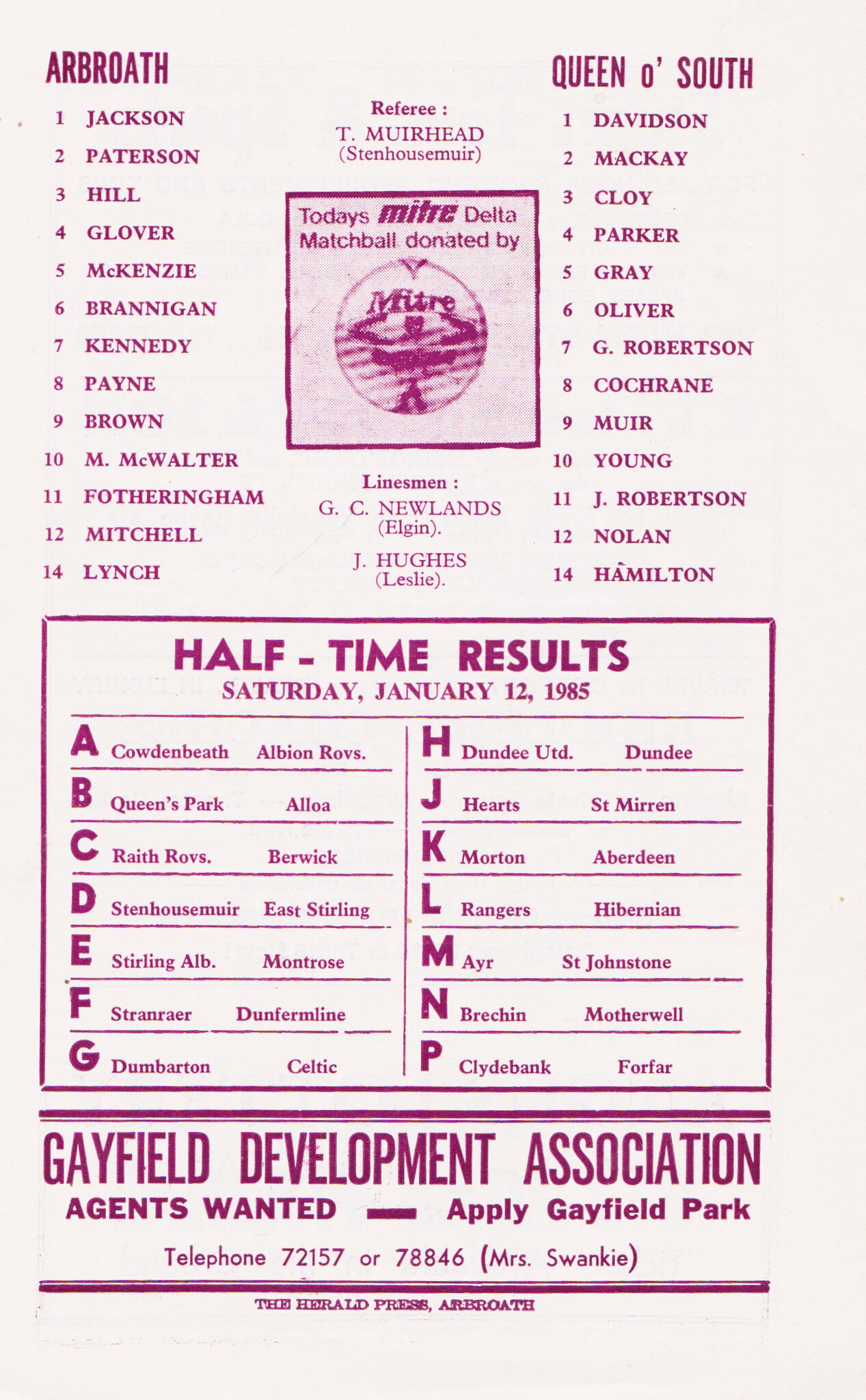This photograph features halftime results presented on a light pink background with dark pink to purple text. At the top left, it lists "Arbroath," followed by the names of their players: Jackson, Patterson, Hill, Glover, McKenzie, Brannigan, Kennedy, Payne, Brown, M. McWalter, Fotheringham, Mitchell, and Lynch. In the top right, it features the opposing team "Queen of the South" with players: Davidson, McKay, Cloy, Parker, Gray, Oliver, G. Robertson, Cochrane, Muir, Young, J. Robertson, Nolan, and Hamilton.

Prominently centered is a square box with text referring to the match officials and sponsor, reading: "Referee T. Muirhead, Stan Halsmuir, Today's Mitre Delta match ball donated by Mitre." Beneath this, in smaller text, it mentions the linesmen: "Linesman, G.C. Newlands, Elgin, J. Hughes, Leslie."

The document further details the halftime results from Saturday, January 12, 1985, presented in a purple box with alphabetized columns from A to G on the left and H to P on the right. Teams included are Calden, Beeth, Albion Rovers, Queens Park, Alloa, Raith Rovers, Berwick, Stenhousemuir, E. Stirling, Stirling, Arbroath, Montrose, Stranraer, Dunfermline, Dumbarton, Celtic, Dundee United, Dundee, Hearts, St. Mirren, Morton, Aberdeen, Rangers, Hibernian, Ayr, St. Johnstone, Brechin, Motherwell, Clydebank, and Forfar.

A horizontal purple line separates the bottom section that reads: "Gayfield Development Association, Agents Wanted. Apply Gayfield Park, Telephone 72157 or 78846, Mrs. Swanky." Finally, the document credits "The Herald Press, Arbroath" at the very bottom. The overall color scheme maintains a cohesive light pink with dark purple text, providing a nostalgic and clear presentation of the halftime details.